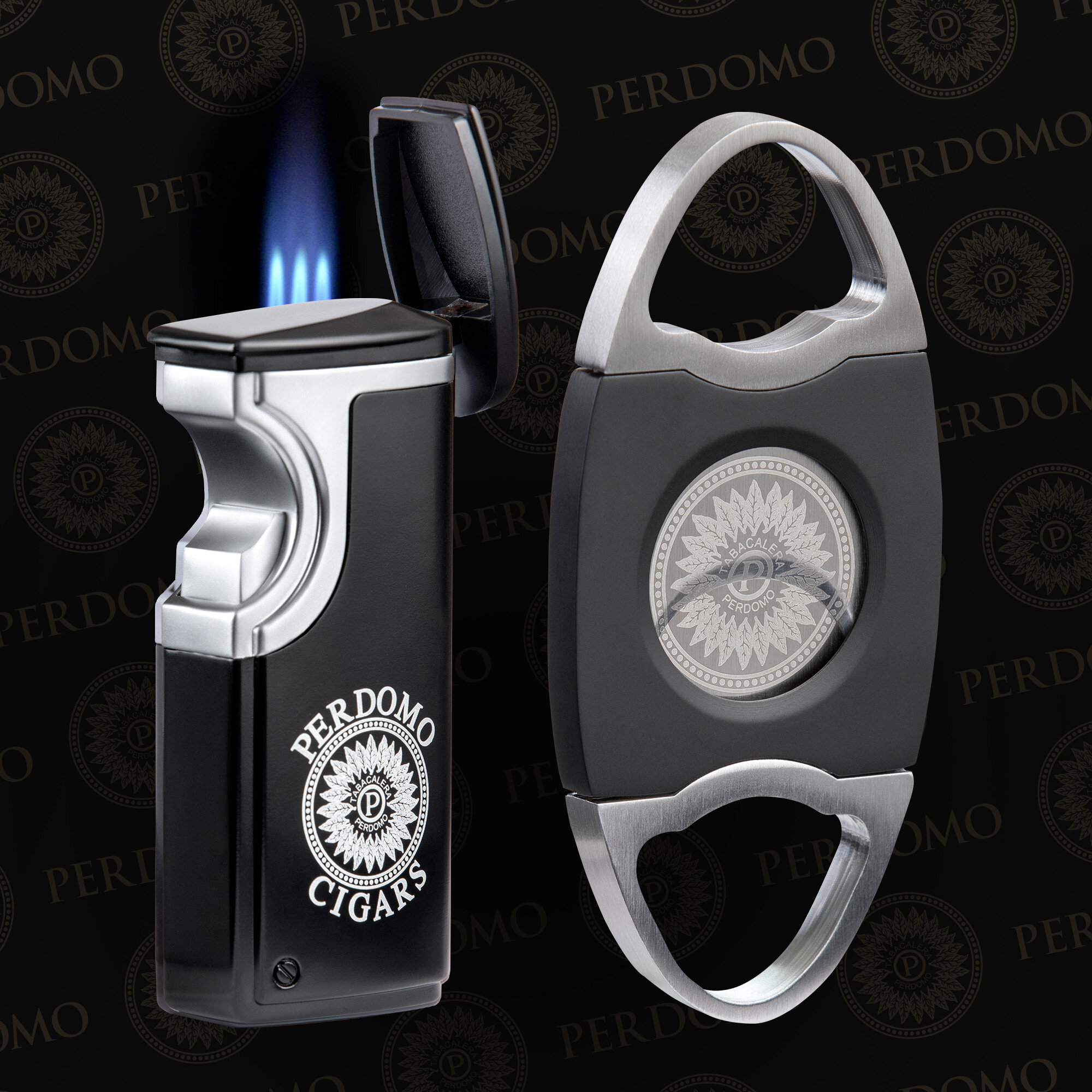This photograph features two sleek smoking accessories against a black background adorned with a transparent watermark reading "P-E-R-D-O-M-O." The primary focus is a sophisticated black and silver butane lighter on the left. The lighter boasts a shiny black case with silver metallic accents. Its lid is flipped open to reveal a robust blue butane jet flame. The lighter features a semicircular silver ignition switch that fits a thumbprint comfortably. The base of the lighter prominently displays the text "Perdomo Cigars" along with the Perdomo logo, which consists of a circular design resembling a sunflower with an interior circle containing a 'P' and the words "Tabacalera Perdomo."

Adjacent to the lighter, on the right, is an elegant oval-shaped cigar cutter. Like the lighter, the cutter is two-toned in black and silver. It has a dark gray center flanked by two sturdy silver handles. The Perdomo Cigars emblem is also prominently displayed in the middle of the cutter. The functional design of the cutter includes two openings at the top through which the cigar is inserted for a precise cut.

Together, these items create a visually appealing arrangement that highlights the craftsmanship and brand identity of Perdomo Cigars.